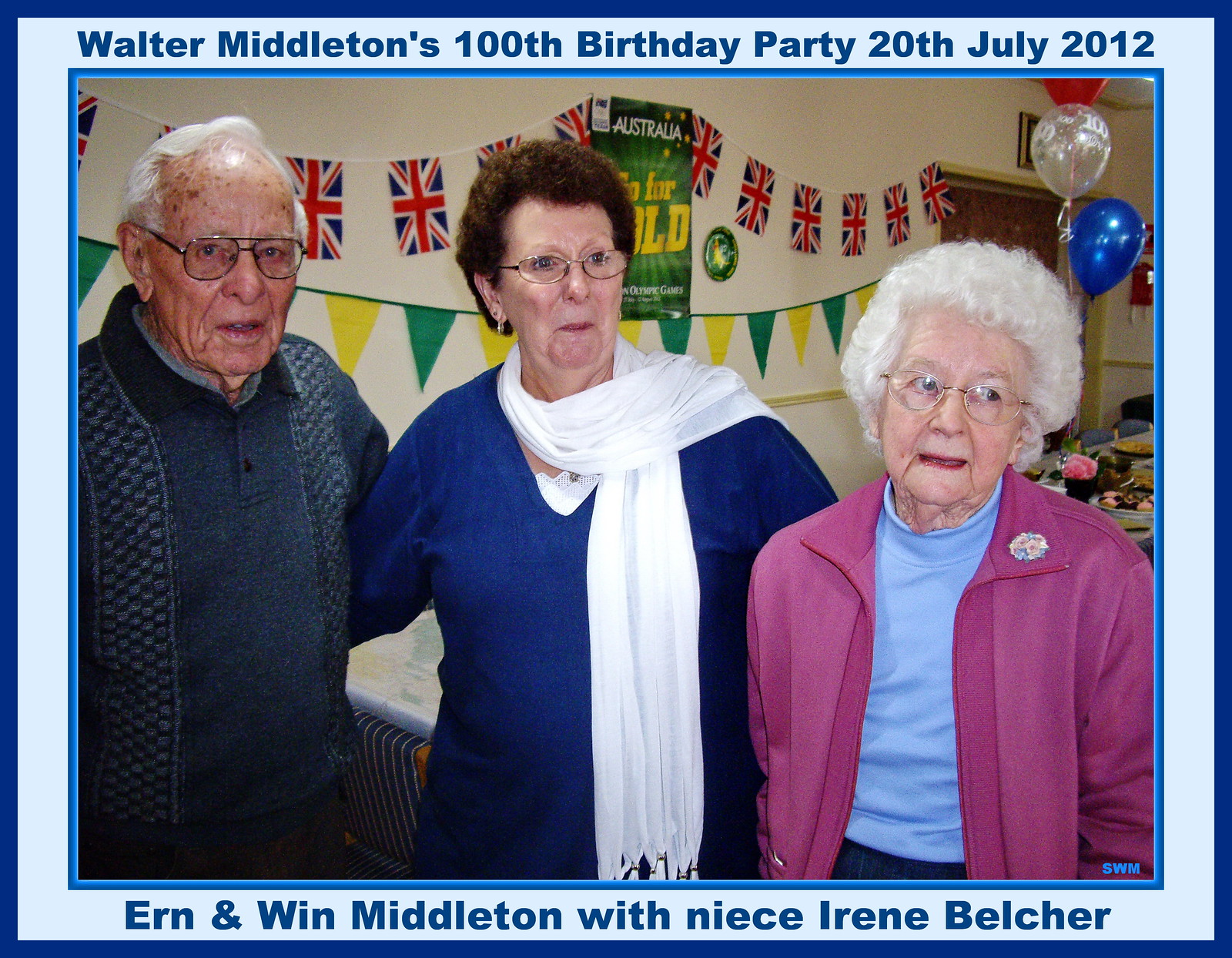The image is a digitally framed photograph featuring a celebratory event with a backdrop adorned with strings of flags, including the Union Jack, and posters, including one that says "Australia." The photo is bordered by a three-tiered, digital frame comprising a thick blue outer line, an even thicker light blue area with text, and a medium blue inner line surrounding the picture. The top text reads in navy blue, "Walter Middleton's 100th birthday party, 20th July 2012," while the bottom text indicates, "Earn and Win Middleton with niece Irene Belcher."

Within the photograph, three individuals are shown standing and embracing each other. On the far left is Earn Middleton, an elderly man with white hair, wearing glasses. In the center is the younger niece, Irene Belcher, dressed in a blue sweater with a white scarf, wearing glasses, and sporting short, dark hair. To the right is Wynne Middleton, an elderly woman with white hair and glasses, donning a lavender jacket over a light blue mock neck, adorned with a pin on her left lapel. Also visible in the image are colorful birthday elements such as red, white, and blue balloons and what appears to be food. The photograph captures a moment of familial celebration, displaying a rich array of colors including blue, pink, green, yellow, and black, reflecting the joyous nature of Walter Middleton’s centenary celebration.